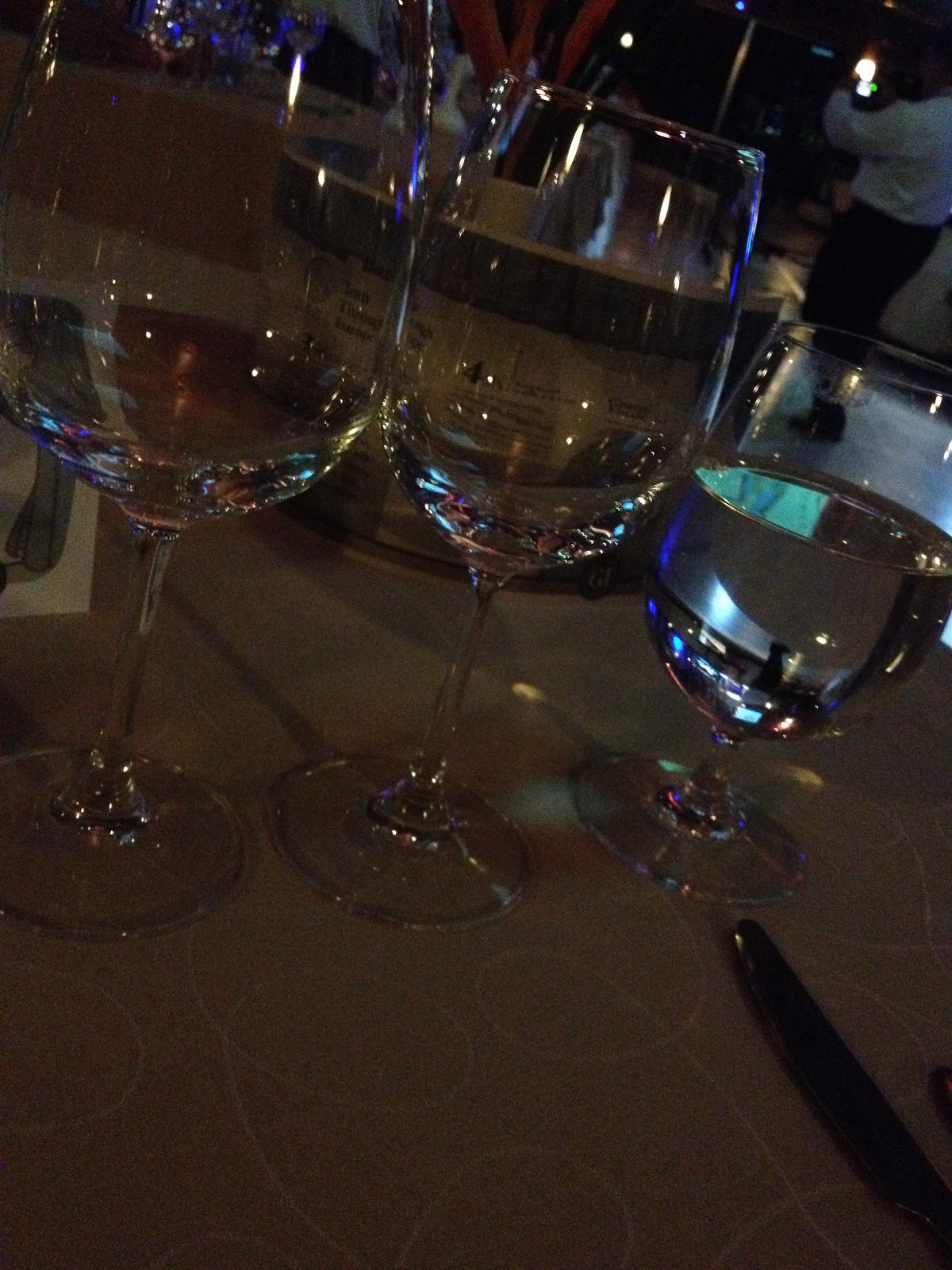In a dimly lit room, three elegant glasses are centrally arranged on a dark table, creating a striking visual contrast against the shadows. The ambient lighting is minimal, with faint lights in the upper right-hand corner softly reflecting off the glasses and casting delicate patterns. Two of the glasses are tall with long stems and rounded bottoms, while the third is a shorter, similarly shaped version, maintaining the set's cohesive aesthetic. All three glasses contain a clear liquid, possibly water or a transparent alcohol, enhancing their reflective quality. A menu or piece of paper is discernible on the table's left side, adding context to the setting. A mysterious, dark utensil—likely a pen or knife—rests in the bottom right corner. The scene is completed by the partial figure of a man dressed in a white long-sleeved shirt and black slacks, standing in the background. A container holding various bottles is also visible, blending into the intricate, low-light ambiance, which highlights the intricate, curvature design of the tablecloth underneath the glasses.